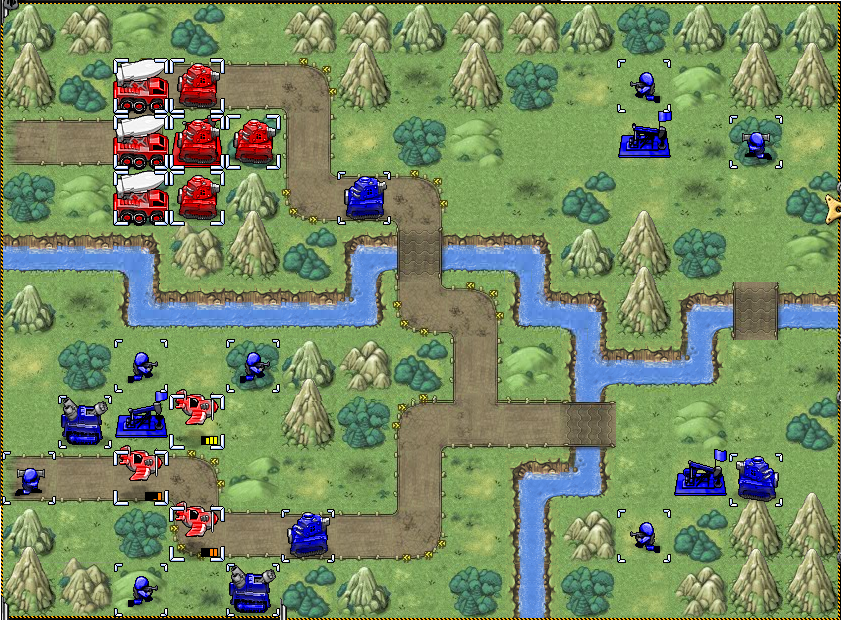The rectangular image, framed with a thin brown border, depicts an outdoor scene reminiscent of an old video game or a basic mobile game's screenshot. The setting is a lush, cartoon-like environment with ample green grass, various trees, shrubs, mountains, and hills. A river or stream winds through the landscape, crossed by several bridges. The image is divided into opposing teams, highlighted by their solid red and solid blue colored tanks, trucks with missile attachments, and planes. The teams appear to be engaged in tactical combat, with the blue team positioning several infantrymen—seven in total—crouching and aiming their weapons from the shrubs. Red vehicles and blue vehicles are scattered across the map, with some stationed at strategic points and others on pathways. This detailed scene is devoid of any textual elements, focusing entirely on the strategic placement and interaction of the combat units in a vividly digital battleground.